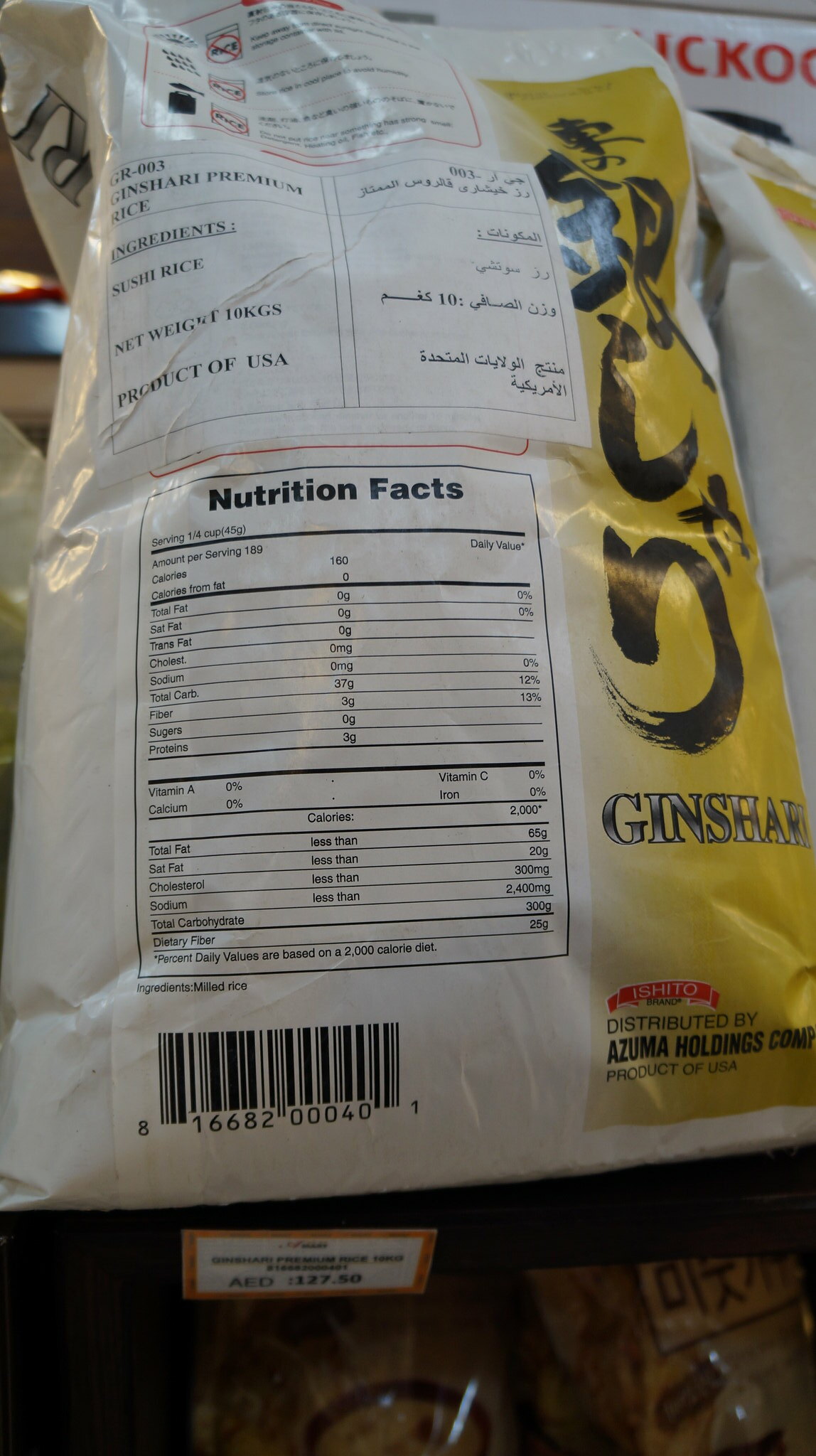This detailed image captures the back of a chip bag package, prominently featuring a Nutrition Facts box located at the bottom center. Below this nutritional panel, there's a barcode stamped, numbered 1668200040. Above the Nutrition Facts, an ingredients list specifies sushi rice, detailing the weight and the origin of the product. The right section of the packaging is adorned with black calligraphy against a light green background, with additional elements of Chinese writing present.

The manufacturer's information reveals the brand name "Genshack" or "Genshacky," and the item is distributed by Azuma Holdings Company. The bag displays a distinct color pattern; the left portion is white, transitioning to yellow on the right. There's a notable red banner towards the bottom right with the text "S-H-I-T-O."

Captured on a store shelf, this package has a small brown-outlined white sticker affixed to its front, typical of retail environments. The visual composition includes a mix of Asian-inspired graphics and writing, providing a cultural touch to the packaging.